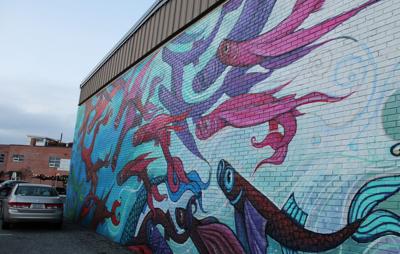The photograph showcases the side of a building adorned with a vibrant mural painted in a graffiti style. The mural predominantly features an array of colorful fish that appear to be swimming underwater. These fish range in colors from pink-ribbed creatures with shrimp-like textures to crimson fish with blue and purple flowing ribbon-shaped fins. The mural also incorporates playful elements like smiley faces and colorful swirls, especially concentrated on the right-hand side, which is washed with hues of teal and white.

The building, constructed of red brick, is positioned at a slight angle to the left. Alongside the mural, a parking lot can be seen, with a small van parked near the building. In the background, part of the city skyline and another smaller red brick building are visible, adding depth to the urban setting of the photograph.